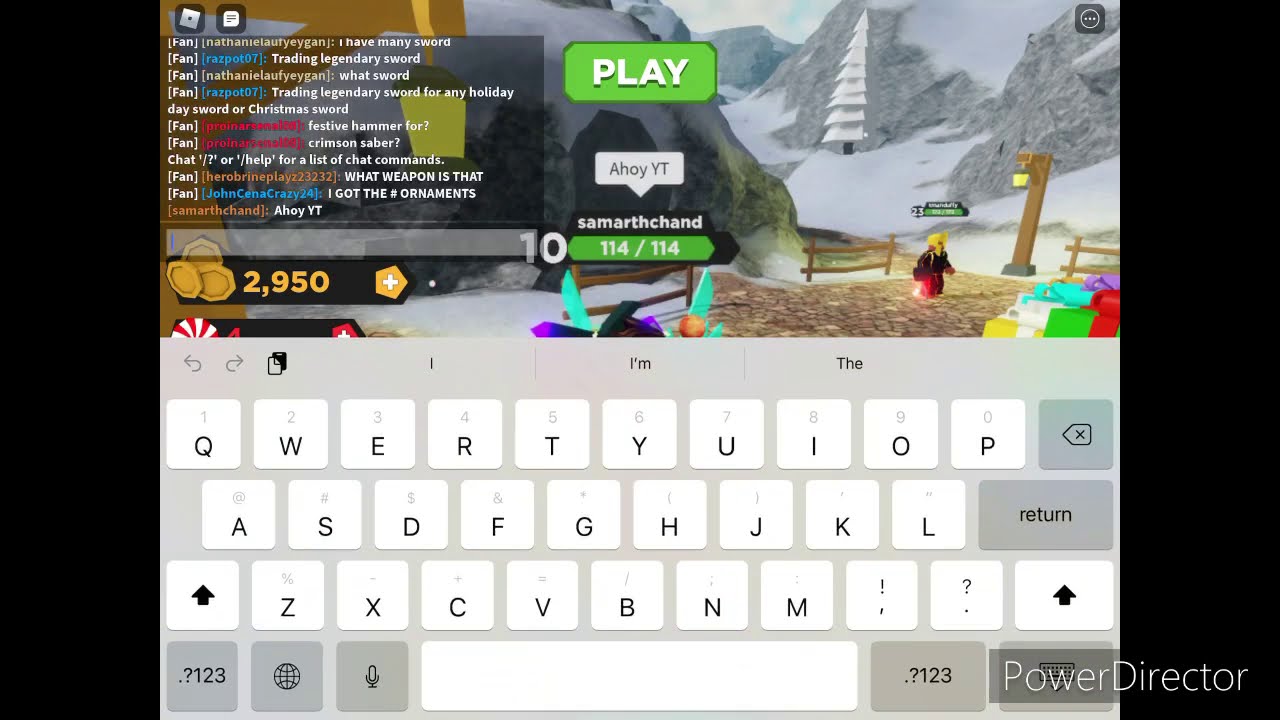In this detailed screenshot of a mobile video game, the top half of the image showcases a fantasy scene where a small character with blonde hair, dressed in a black top and red skirt, walks along a cobblestone path through a snowy mountain landscape adorned with snow-covered trees and scattered Christmas presents. The central upper part of the screen features a green rectangular "PLAY" button with white lettering, situated above the player’s username, Samantha Tand, indicating her ranking as 114 out of 114. A live chat runs along the left side, containing messages such as “I have many sword, trading legendary sword,” alongside a display of in-game coins totaling 2,950. The lower half of the image is dominated by a virtual QWERTY keyboard with light and dark grey keys, set against a grey background, typical of an Apple device's keyboard layout. Notably, the word "PowerDirector" is printed in white in the bottom right corner. The scene is framed by black borders on both sides, emphasizing the focus on the gameplay and keyboard interaction.